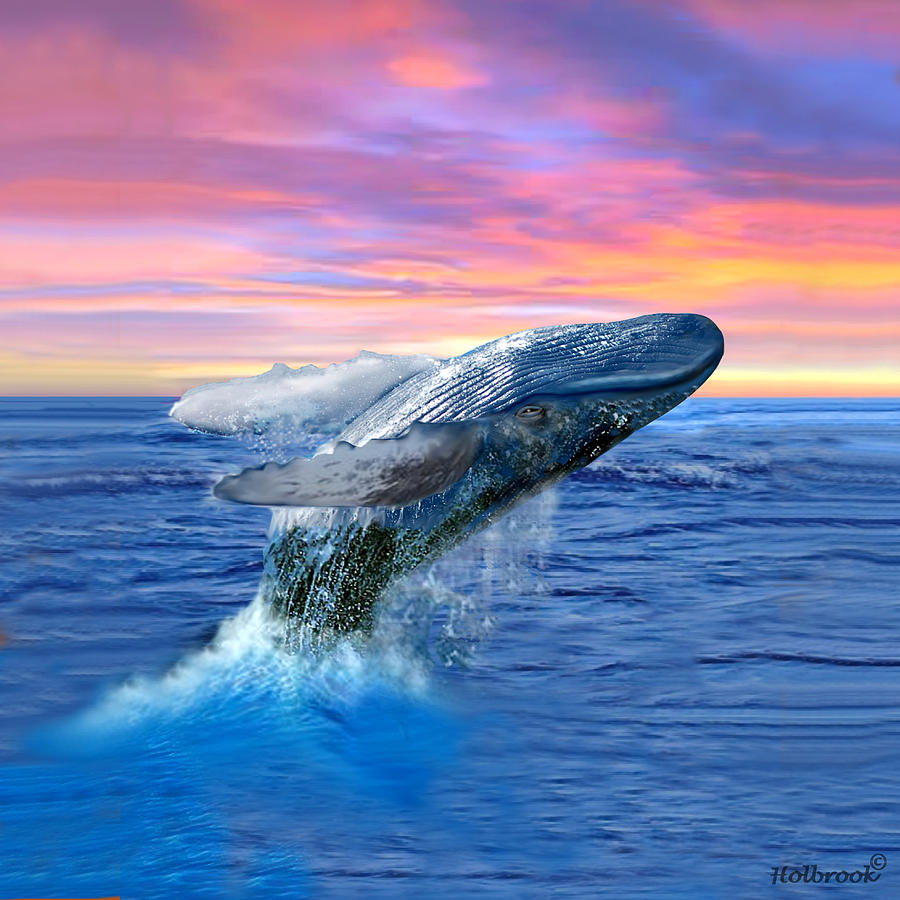This is an artistic depiction of a whale, prominently featuring a photorealistic blue whale diving backwards into a vibrant navy blue ocean. Water ripples out near its tail in shades of white and blue, with droplets glistening off its back and near its fins. The whale's body is a blend of blue and greenish hues, and you can see its eyes gazing upwards as it breaches, almost as if performing a backflip. The background sky is an exquisite tapestry of colors, transitioning from pink, golden, and orange to yellow, reminiscent of an amber night sky at sunset or sunrise, with hints of blue from the sun's outer edges. The ocean below is clear and luminous, saturated in a bright blue. In the lower right corner, the artist's or photographer's trademark "Holbrook" is visible, accompanied by a copyright symbol. The artistic style combines photorealism for the whale with a more illustrated approach for the ocean and sky, giving the image a unique and captivating visual contrast.